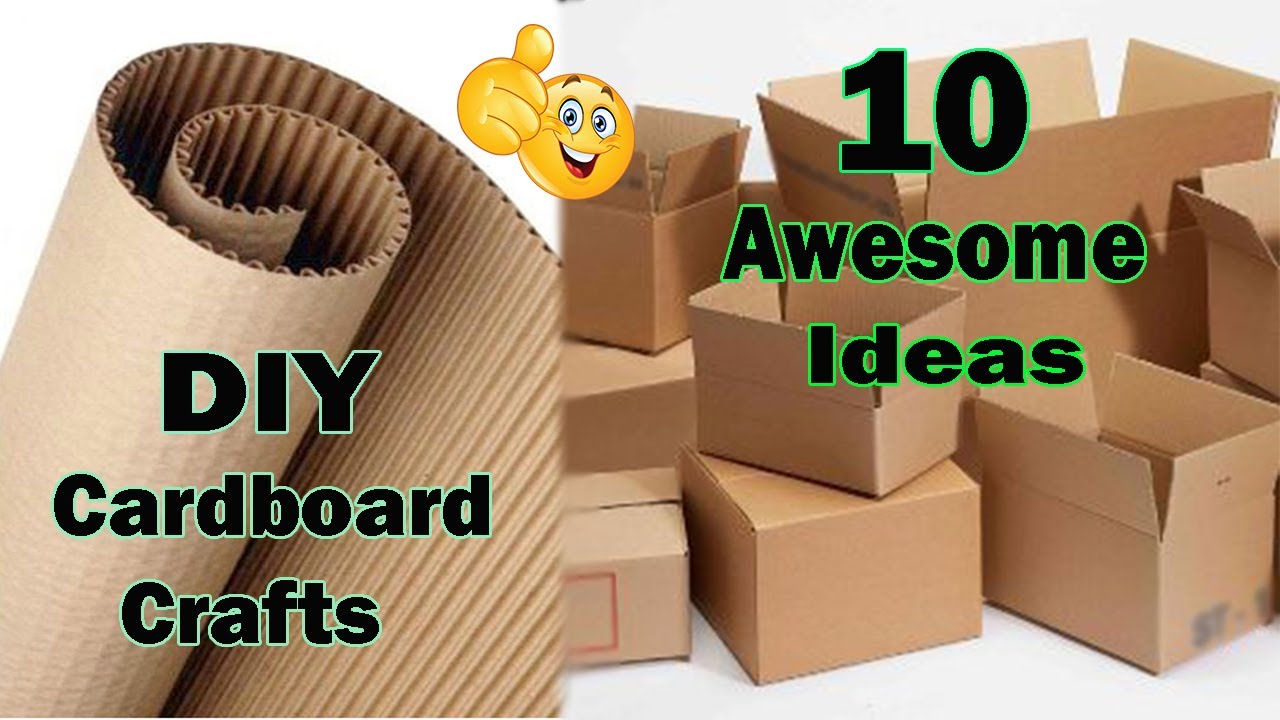The image features a split design highlighting DIY cardboard crafts. On the left side, there is a roll of corrugated cardboard with a wrinkled effect, accompanied by the title "DIY Cardboard Crafts" in black text edged with pistachio green. On the right side, a collection of cardboard boxes in various sizes, some open and some closed, is displayed with the text "10 Awesome Ideas" in black font with a green outline. Centrally placed between these elements is a smiley face emoji giving a thumbs up, adding a touch of fun to the informative image. The image appears slightly blurry in the middle but overall effectively showcases creative uses for cardboard.